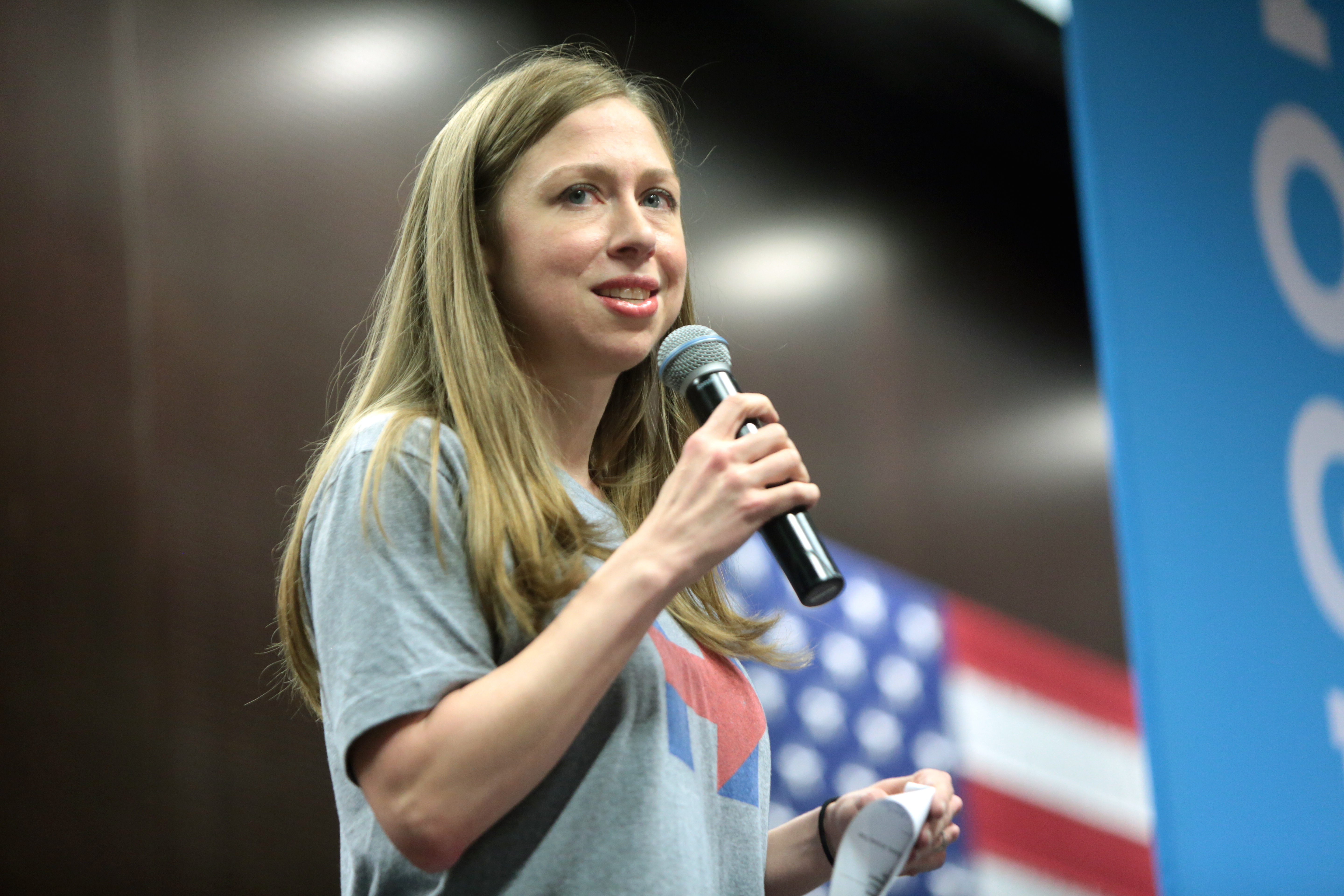The image features Chelsea Clinton standing on stage delivering a speech. She is holding a handheld microphone close to her mouth with her right hand while her left hand grasps a folded piece of paper, possibly a script. Chelsea has long, sandy brown hair, and a light complexion, and she's wearing a gray short-sleeved t-shirt adorned with her mother's campaign logo, a blue "H" with a red arrow pointing to the right. She appears to be smiling slightly and is looking off to the side, perhaps engaging with an audience member. On her left wrist, she wears either a bracelet or a watch. The photograph has a professional quality with a blurry background. In the backdrop, an American flag is visible along with a blue and white vertical banner with unreadable text. The setting appears bright due to good lighting, likely capturing a moment from the campaign trail of Hillary Clinton from a few years ago.